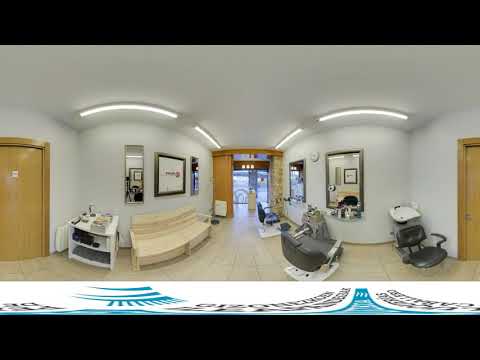The image depicts an interior shot of what is likely a hair salon or a waiting area, potentially resembling a hospital lobby due to its sterile and meticulously organized appearance. The room is spacious with white-painted walls and a white ceiling, illuminated by long strip lights that run near the edges. Several mirrors are mounted on the walls, with three being prominently mentioned. There are multiple sinks, typically seen in a hair salon, along with leatherette chairs that seem adjustable for reclining, indicating their use for hair treatments. 

Towards the far end of the space, a glass door leads to the outside, and near this door could be a receptionist desk. The floor is covered in beige tiles, adding to the clean and professional look. On one side, there is a wooden bench in front of windows on the left, accompanied by a white table cluttered with unspecified items. In the middle of the room, there is a white clock mounted on the wall, ensuring visitors can keep track of time.

Additional seating is provided by several black chairs with white bases, likely designated for waiting guests. A small white cabinet or table is located on the lower left side of the image, and a white garbage can provides for cleanliness. On the left wall, between the windows or booths, there is what seems to be a map or a picture, although its details are indistinct. Notably, brown doors are situated on either side of the image, contributing to the overall organized partitioning of the space. The image's perspective suggests some distortion, probably from being captured by a 360-degree camera, giving a slightly curved appearance to the walls and fixtures.